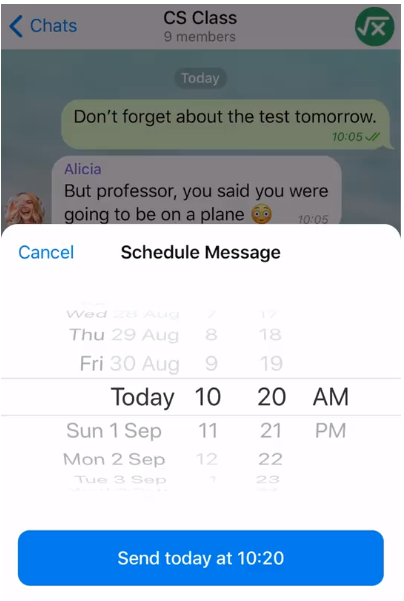This is a detailed screenshot of a messaging application, specifically featuring a group chat for a computer science class. 

At the very top of the screen, there is a faintly muted square, partially obscured. A white rectangle spans the entire width of the top, with a blue left-pointing arrow resembling a sideways "V" on the far-left side. Next to the arrow, the word "Chats" is displayed in blue text. Centrally located in bold black text is the title "CS Class," indicating the group chat's subject. Directly beneath this title, is a smaller, non-bolded black text stating "9 members" to denote the group size. On the far-right side, a green circle displays an icon with a division sign overlaid atop an "X."

The main content is set against a green background. At the top of this section, inside a green oval, the word "Today" is displayed in white text. Below this, a series of message bubbles are shown. The first message bubble, with a green background and black text, reads: "Don't forget about the test tomorrow." 

The subsequent message bubble has a white background. In the upper left-hand corner of this bubble, "Alicia" is written in gray text, and below, in black text, it reads: "But professor, you said you were going to be on a plane" followed by a scared face emoji.

Further down the screen, there is a white square containing blue text that reads "Cancel" in the upper left-hand corner. Centered within this square, in bold black text, are the words "Schedule Message." Accompanying this is a wheel interface that allows for the selection of the day, date, month, and time. The selected option in the center, highlighted with a light gray line above and below it, reads "Today 10:20 AM."

At the very bottom of the screen, a prominent blue rectangle contains the text "Send today at 10:20" in white.